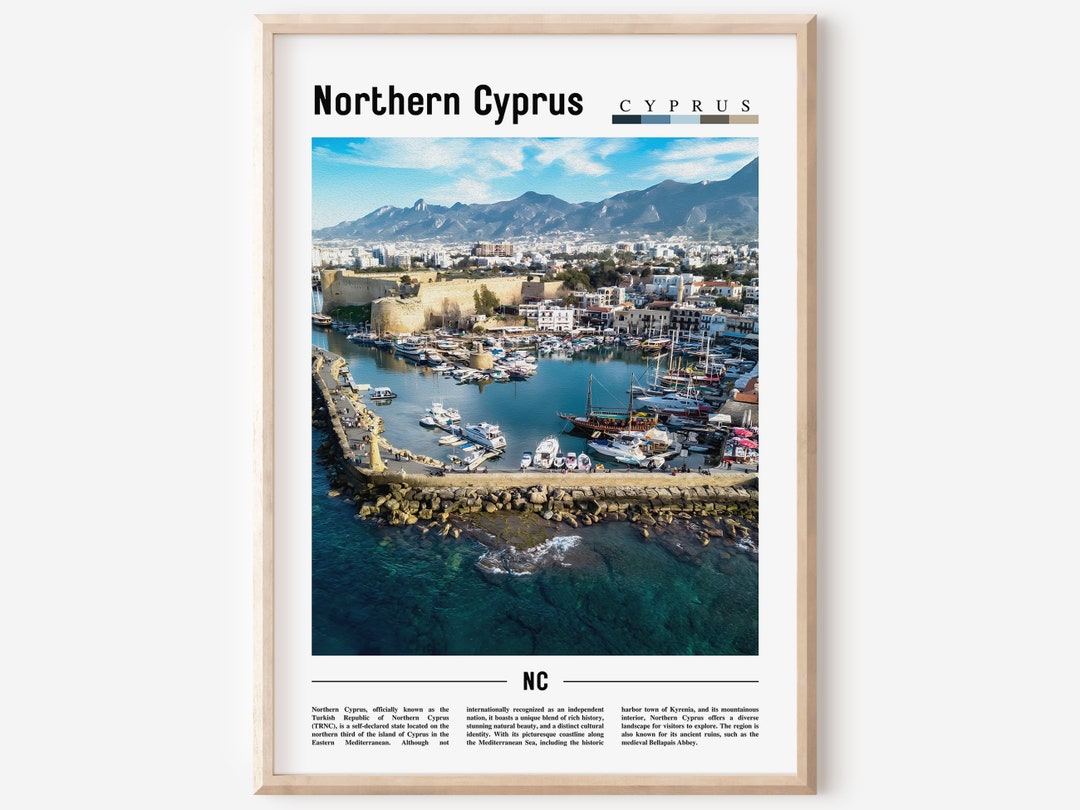The image is a full-color, square photograph taken outdoors on a sunny day, using natural light. It features a clean, light gray background with no border. At the center of the image is an unpainted, unvarnished wooden frame containing a white background. Within this frame, the words "Northern Cyprus" appear in bold black font, followed by the word "Cyprus" in a slightly smaller black font. Below these words is a small, thin rectangular border with color swatches in shades of black, light blue, dark blue, pink, and brown. 

The main photograph showcases the city of Northern Cyprus, set against a backdrop of rolling hills and low mountains. The sky is adorned with puffy clouds, and the day is visibly clear and bright. The city is surrounded by exceptionally clear water, featuring a marina with numerous docks and boats. The urban landscape includes several buildings, a large stone walkway, a road, and various boulders. There are also green trees indicating a temperate, mild climate. At the very bottom of the photograph, there is a line of text that is too small to read, likely containing additional information about Northern Cyprus.